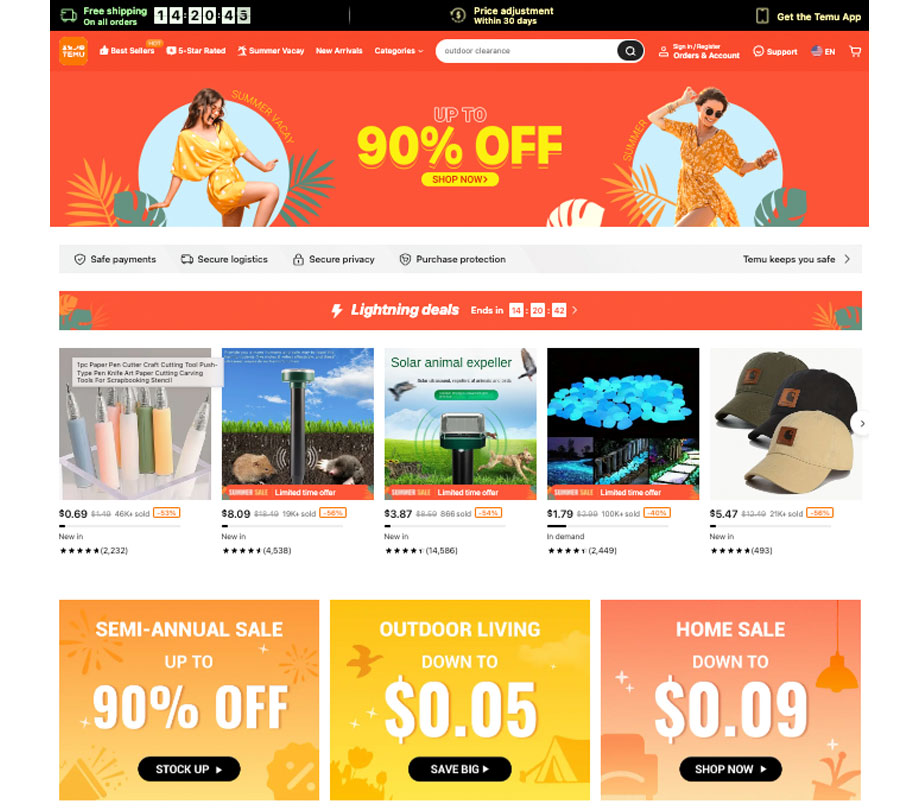Here is a cleaned-up and detailed caption for the image described:

---

The Teemo webpage is visually divided into three distinct sections. The top section, dominated by a vibrant orange color, features a prominent 90% off discount message with a "Shop Now" call to action. Accompanying this, there are two women happily flouncing about in summer dresses. A countdown timer at the top of the page, set at 14 hours, 20 minutes, and 43 seconds, emphasizes the limited-time nature of the free shipping offer on all orders.

In the middle section, key features of the shopping experience are highlighted: "Safe Payments," "Secure Logistics," "Secure Privacy," and "Purchase Protection." This part assures customers of the site's reliability and security.

The bottom section showcases the "Lightning Deals," which are also tied to the same countdown timer. Among the deals available are eyebrow zappers at 10 for 69 cents, a solar animal expeller designed for pest control, and some unidentified affordable gadget. Additionally, there are ball caps priced incredibly low.

Finally, the very bottom section advertises the Semi-Annual Sale, featuring categories like "Outdoor Living," with items starting as low as five cents, and the "Home Sale," with prices beginning at nine cents. This sale also boasts a significant 90% discount.

---